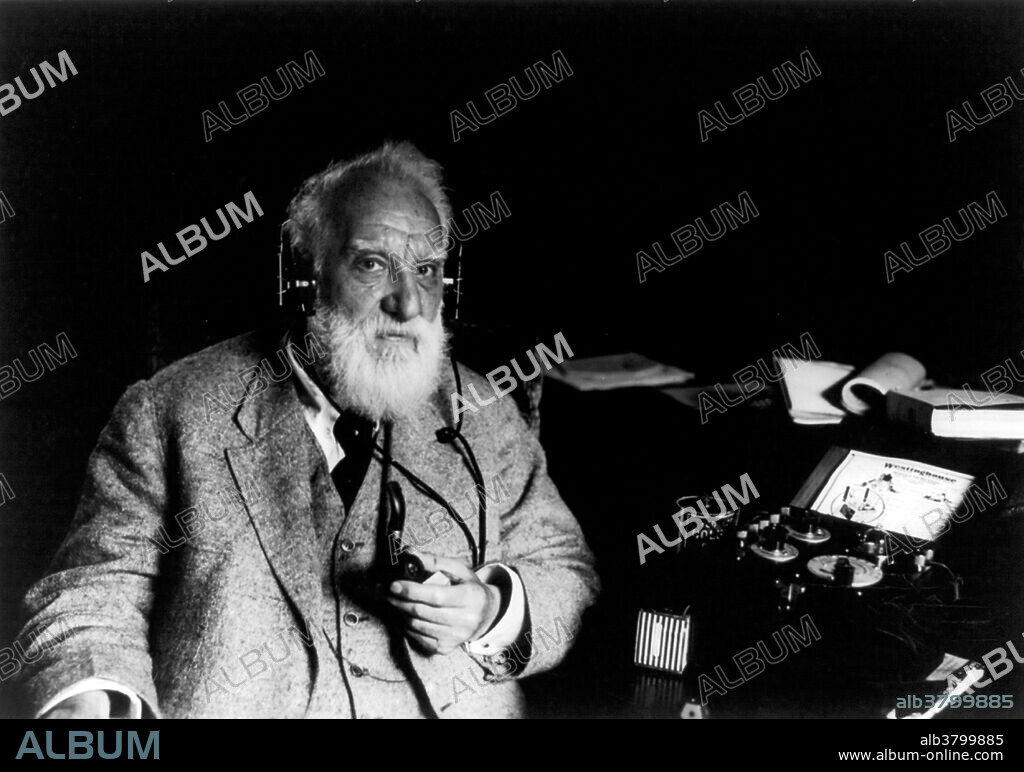This is a detailed black and white photo of an older gentleman, approximately 70 years old, with thick, all-gray hair and a robust beard and mustache. His dark eyes and medium complexion give him a distinguished appearance. He is dressed in a light-colored suit, complete with a white button-down shirt, a black tie, and a gray wool tweed suit jacket and vest. He is holding a black tobacco pipe in one hand and a microphone that hangs down to his chest in the other. Large, black, metal headphones cover his ears, with wires trailing down and resting on his chest. In the background, there's an instrument resembling a recording device or music apparatus with three round knobs, a dial, and additional wires attached, indicating a technological setup. Behind him, a cluttered desk with books and papers can be seen. The image features multiple instances of the word "album" and displays a website, www.album-online.com, suggesting a promotional context. The overall aesthetic and the man's attire hint at a vintage era, perhaps from the 70s or 80s.